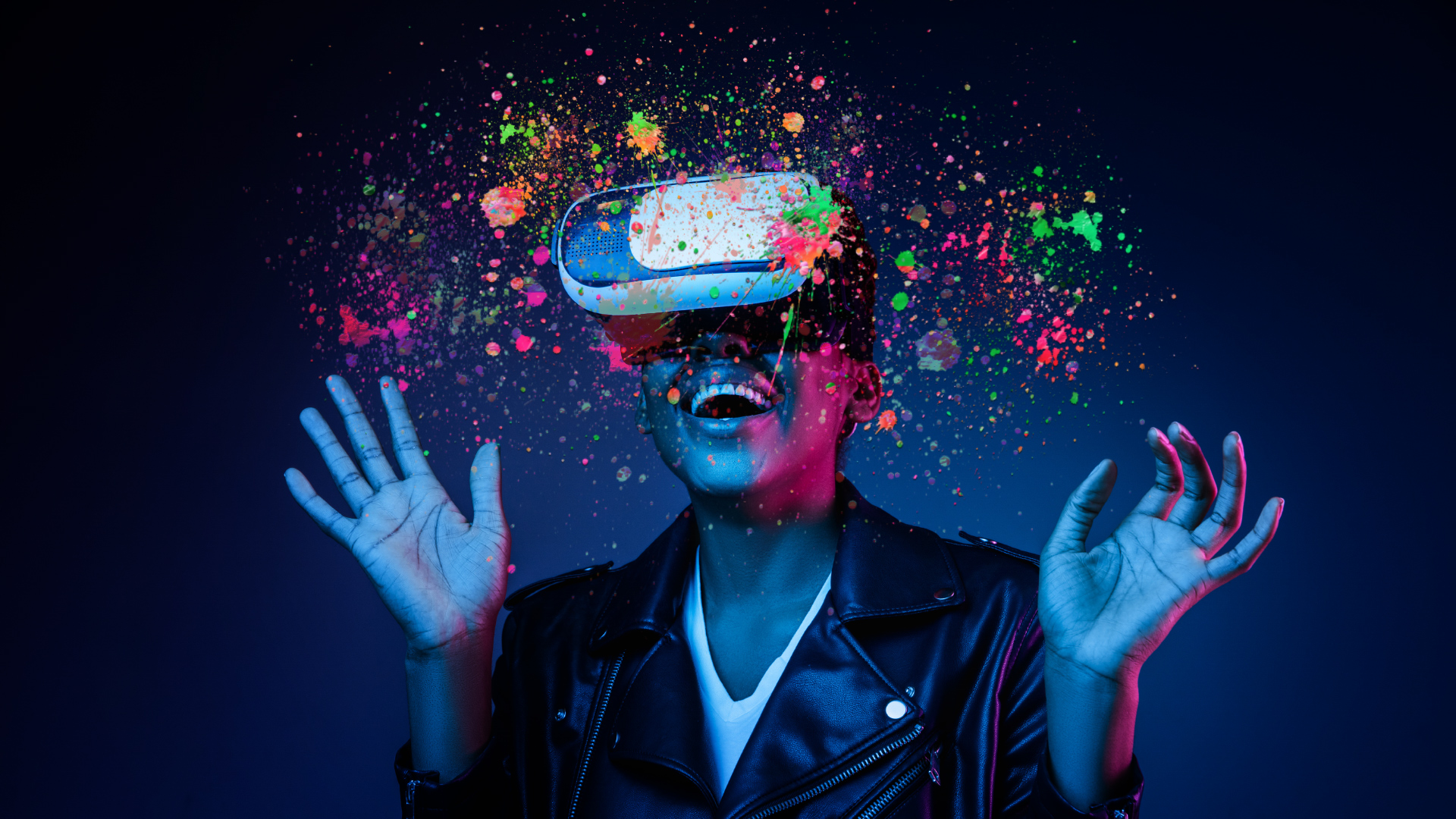The advertisement image features a woman with darker skin, energetically posed with her hands raised and head tilted slightly to the upper left, embodying the thrill of the virtual reality experience. She wears a stylish black leather biker jacket adorned with diagonal zippers, paired with a white V-neck t-shirt. Her bright white teeth are visible in a large, joyful grin. The setup includes a blue-toned, high-contrast background with hints of pink, creating an electrifying, neon ambiance. The scene is digitally enhanced, likely passed through editing software like Lightroom, to emphasize textures and vibrancy. Over the scene are vibrant splashes of green, pink, and orange paint, visually representing the stimulating world she's immersed in via her VR headset. A pin on her jacket adds a subtle, personalized touch to her appearance.